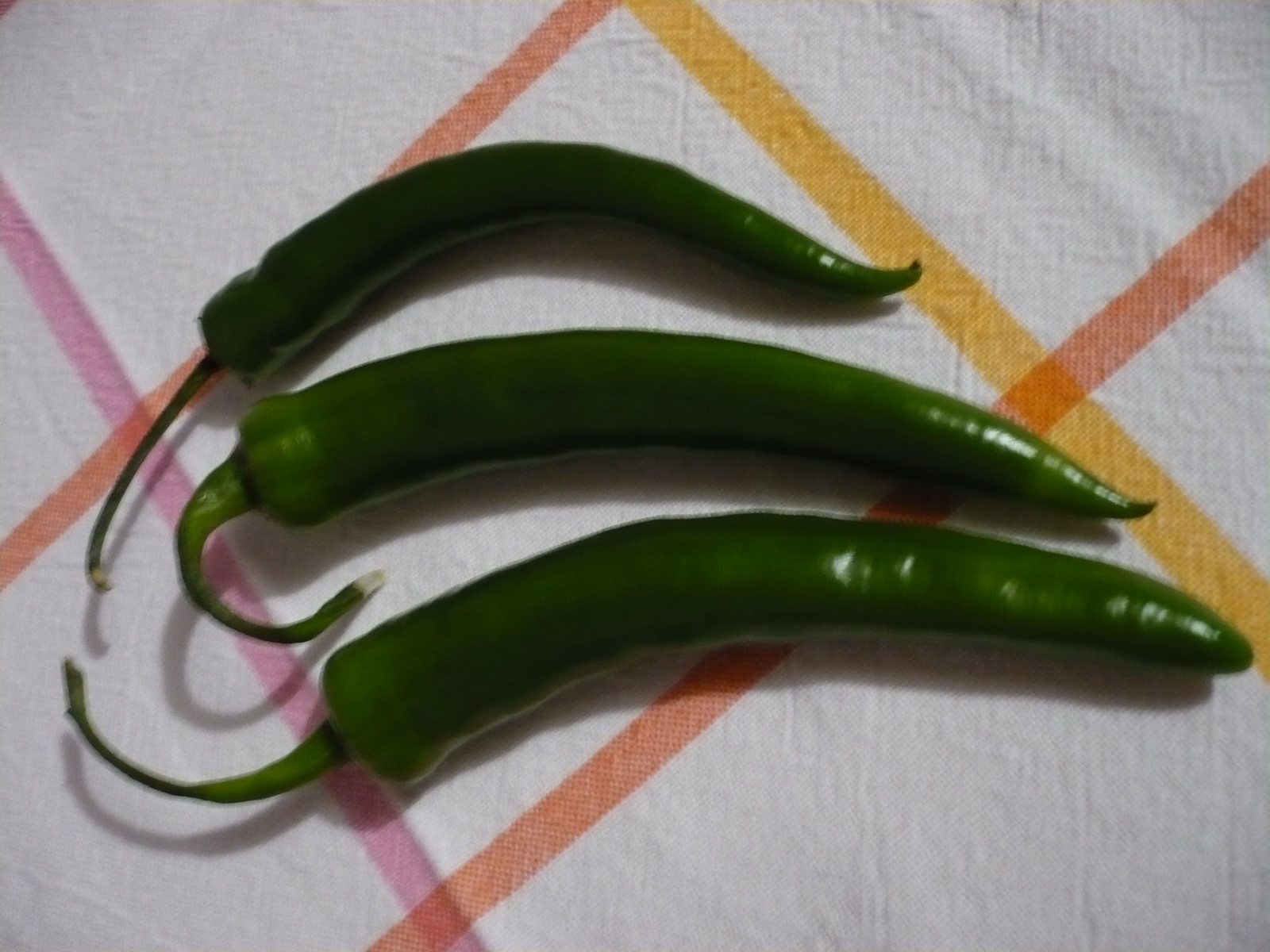This image showcases three green chili peppers arranged horizontally on a white cloth with a checkered pattern in pink, orange, and yellow. The peppers vary in length, with the longest pepper placed at the bottom and exhibiting a slight curve. Above it is a medium-sized pepper with a curled stem, and the topmost pepper is the shortest and most curved, with a straight stem pointing to the left. The organized alignment and the distinct dark green color of the chilies against the vibrant background create a visually striking contrast.